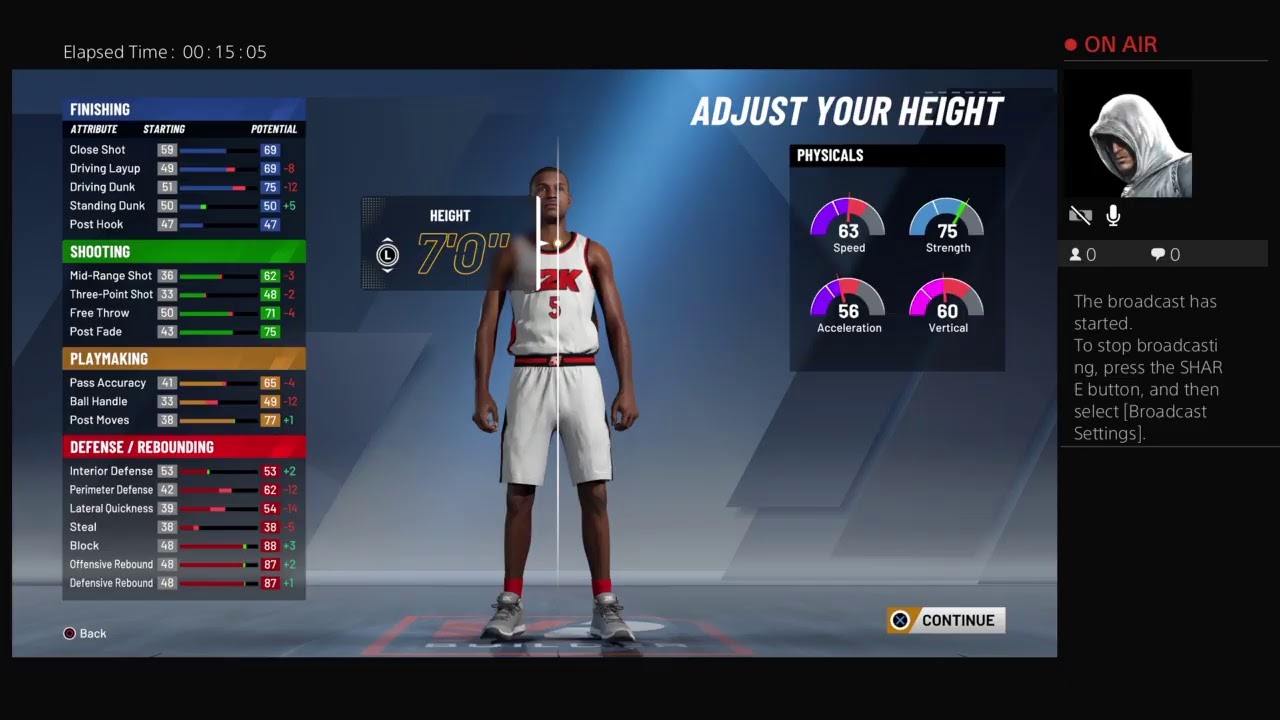The screenshot features a website with a predominantly black background and a blue window occupying about three-quarters of the width. The main focus is an image that appears to be from a basketball game setting. The character showcased is a Black man who looks like a basketball player. He is dressed in a white sleeveless shirt with red writing and the number five on it. His outfit includes long white shorts that go down to his knees, featuring a black and red waistband, red socks, and greyish trainers.

To the right of the image, there is a section titled "Adjust Your Height," accompanied by four car-like dials displaying the numbers 63, 75, 56, and 80 in white. In the upper right-hand corner of the window, there's a picture of a man wearing a grey hoodie, with some text beneath it. The specifics of the text are unclear but suggest a connection to a gaming interface.

The broadcast status is indicated with a message saying, "The broadcast has started. To stop broadcasting, please press the char E button and then select Broadcast Settings." In the upper left corner, there's a lapsed time display showing 00:15:05. Beneath this, there is a large table with several headings, including "Finishing," "Shooting," "Playmaking," "Defense," and an illegible heading that seems to pertain to "Rebounding."

Behind the basketball player character, there is a height indicator showing 70 inches, along with a graphical line passing through his head, suggesting a customizable height feature. At the lower right corner, there's a white "Continue" button, reinforcing the impression of a game settings interface.